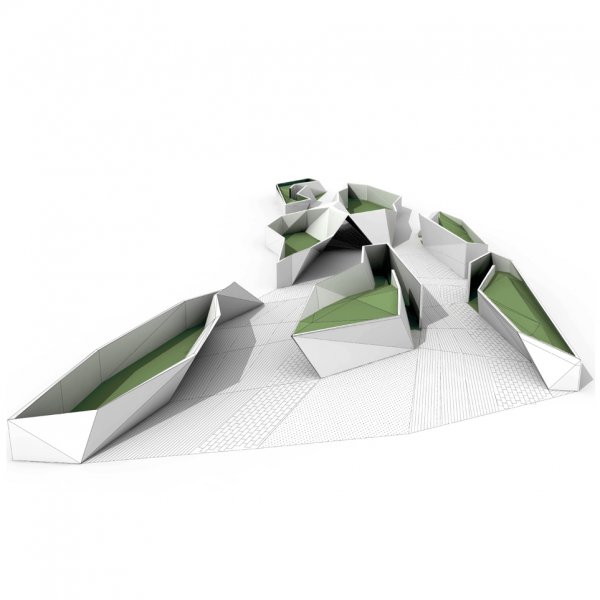The image features a detailed architectural rendering comprising seven distinct, angular shapes with green interiors, resembling secluded, grassy islands or small garden spaces. These shapes, connected by black lines that form a web-like pattern, suggest the form of boats with white surfaces and green inner bases. Gray lines on the ground simulate brick walkways, slightly sloping off into the distance. The rest of the image is characterized by black lines and a white background, enhancing its abstract, architectural quality.